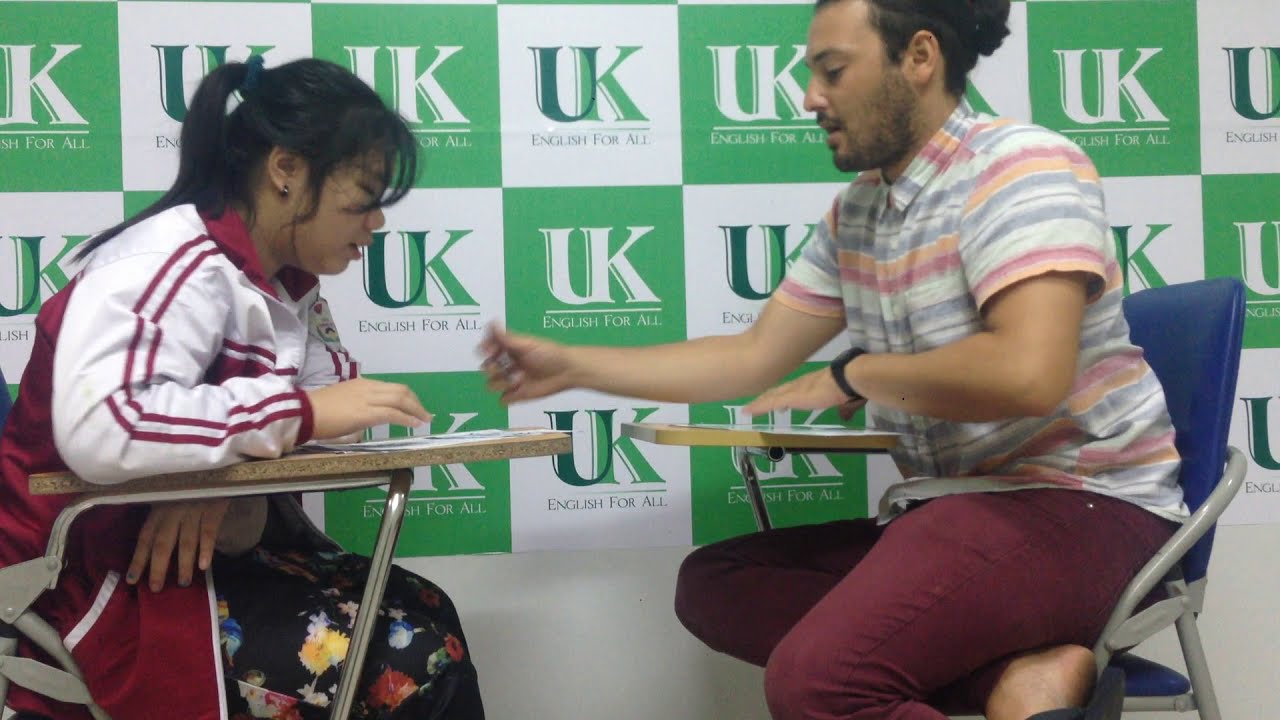In this picture, two people are seated at school desks facing each other, immersed in a moment of concentration. On the right side, an adult man with dark brown hair tied in a bun wears a short-sleeved, collared shirt featuring stripes in hues of orange, blue, pink, white, and purple. He pairs this with long, burgundy red pants and flip flops or slides. He sits cross-legged in a blue chair, extending his hand towards the young woman opposite him. The woman, on the left side of the image, has black hair pulled back in a ponytail and wears earrings. Her outfit consists of a white hooded jacket with red stripes and a floral-patterned black dress adorned with yellow, red, and peach flowers. Both have papers on their wooden desks.

The background features a green and white checkerboard pattern with the text "UK English for All" prominently displayed. The scene suggests an educational setting where the man might be assisting or teaching the young woman.